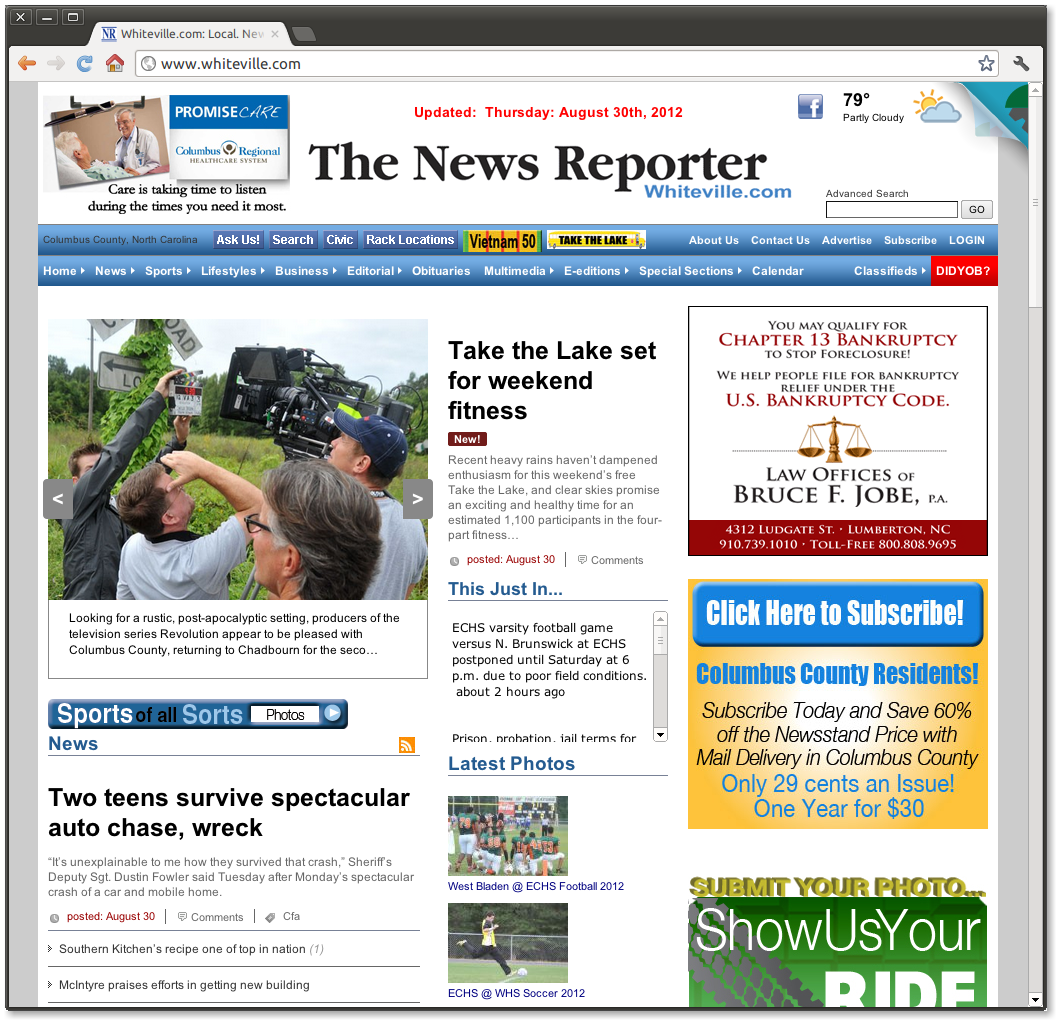**Screenshot from Whiteville.com Newspaper Webpage**

This screenshot captures the webpage for the Whiteville.com newspaper, updated Thursday, August 30, 2012. At the top left corner, there is an image portraying a doctor conversing with an elderly patient in a hospital bed, under the banner "Promise Care, Columbus Regional Health Care System" with the tagline "Care is taking time to listen during the times you need it most."

On the top right, the page displays a Facebook icon, the current weather (79 degrees, partly cloudy), and an "Advanced Search" option. Directly beneath, there is a blue menu bar listing several sections and links including: Columbus County, North Carolina; Ask Us; Search; CMC; RAC Locations; Vietnam 50; Take the Lake; About Us; Contact Us; Advertise; Subscribe; Log In; Home; News; Sports; Lifestyles; Business; Editorial; Obituaries; Multimedia; E-Editions; Special Sections; Calendar; Classifieds; DIDYOB (Did You Observe?). 

The main section includes a photograph of a group of people with cameras captioned: "Looking for a rustic post-apocalyptic setting. Producers of the television series, Revolution, appear to be pleased with Columbus County, returning to Chadbourne for the second...". Adjacent to this, another headline reads: "Take the Lake set for weekend fitness, new. Recent heavy rains haven't dampened enthusiasm for this weekend's free Take the Lake, and clear skies promise an exciting and healthy time for an estimated 1,100 participants in the four-part fitness...". This article was posted on August 30 and has comments.

An advertisement is also present with an image of scales, offering services for filing Chapter 13 bankruptcy to stop foreclosure, provided by the Law Offices of Bruce F. Jobe, PA (contact information included).

Recent updates include a headline for a varsity football game between ECHS and North Brunswick, postponed until Saturday due to poor field conditions, announced about two hours ago. Another news snippet features a story about two teens surviving a spectacular auto chase wreck with a quote from Sheriff's Deputy Sergeant Dustin Fowler. This article was also posted on August 30.

Other content highlights a winning recipe from Southern Kitchen's, McIntyre's praise for efforts in acquiring a new building, and the latest sports photos: Wes Bladen at ECHS football 2012 and ECHS at WHS soccer 2012.

Lastly, there's a subscription offer for Columbus County residents to subscribe and save 60% off the newsstand price, with mail delivery priced at 29 cents an issue, totaling $30 for one year. Additionally, there’s a call for readers to submit their photos and "show us your ride."

---
Since you needed a descriptive and clean caption, I formatted the chaotic voice transcript into an organized and detailed description. The caption retains all relevant information while dividing it into clear sections for easier readability. Let me know if you need further details or adjustments!